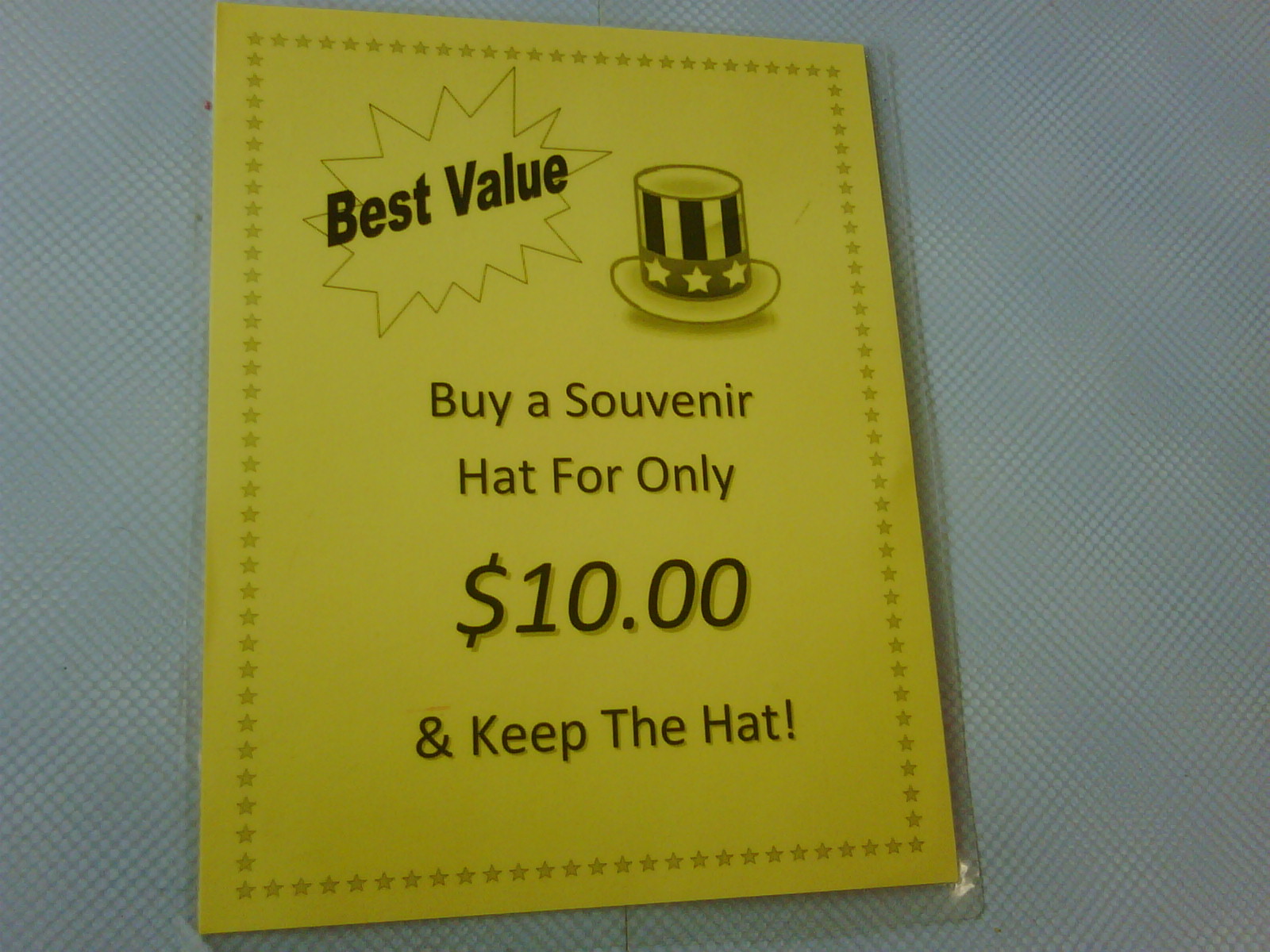This close-up image captures a yellow sign laminated for protection, affixed to a textured white surface. The sign features a grey star-studded border and prominently emphasizes a special offer. In the upper left corner, within a starburst pattern, the words "Best Value" are printed in black. Adjacent to this, to the right, is a black-and-white illustration of an Uncle Sam hat, complete with its iconic red, white, and blue design. The central text boldly announces, "Buy a souvenir hat for only $10," with the price highlighted in larger font. Below this, in a smaller font, it adds, "and keep the hat!" punctuated with an exclamation mark, inviting customers to make a purchase and take the hat home.